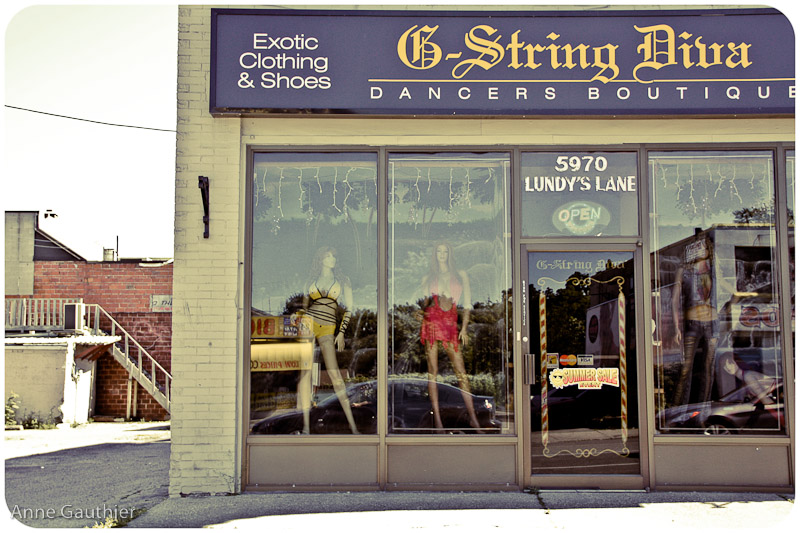The photograph depicts a vintage-style storefront captured with a yellow filter, giving it an old-timey look. In the bottom left corner, a watermark in white text reads "ANNE GAUTHIER," presumably the photographer. The storefront is a single-story, white-painted brick building featuring large glass windows in gray frames and a glass door, also in a gray frame. Above the door, a blue signboard with white text reads "Exotic Clothing and Shoes," followed by "G-String Diva" in yellow text, underlined with a yellow line. Below the line, "Dancer's Boutique" is written in white text. 

The address "5970 Lundy's Lane" is painted in white above the door, which also displays an "open" sign and stickers indicating the acceptance of MasterCard and Visa. The storefront includes three large display windows, each showcasing a female mannequin dressed in different ensembles: the first in a yellow and black costume, the second in a red leather costume, and the third in a blue two-piece costume. Adjacent to the store, on the left, is a small parking lot or alleyway with another small brick building visible in the distance. The overall scene suggests a summer setting, as indicated by a "Summer Sale" sign on the door.